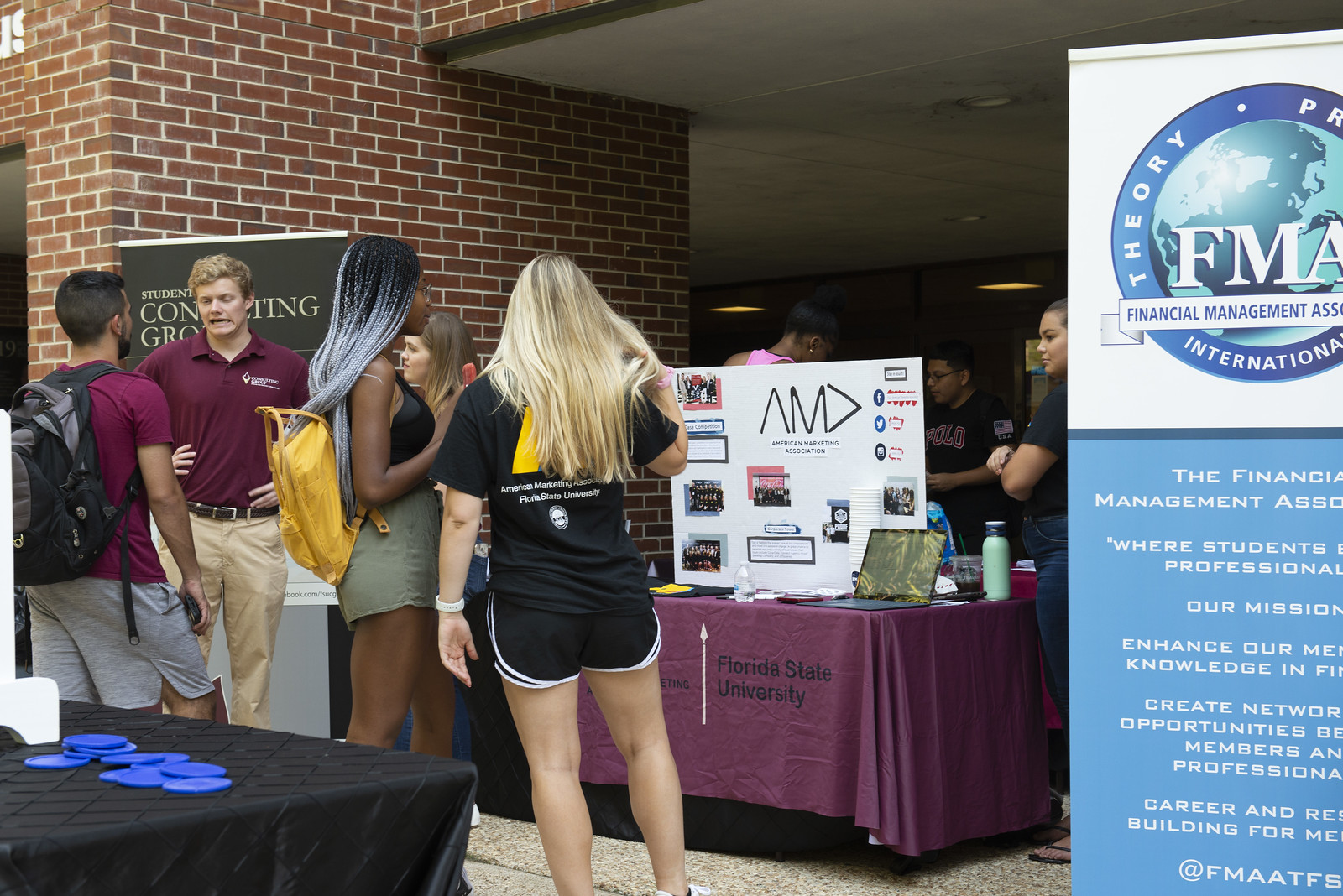In front of a brick building, this color photograph in landscape orientation captures a lively outdoor assembly area, likely the entryway to an auditorium. Central to the image is a table with a red drape emblazoned with the Florida State University spear design. On it, a white poster displays images of student groups, a small water bottle, an open laptop, and various promotional materials. In front of this table stand two young women: an African-American woman with a yellow backpack and olive shorts, alongside a blonde woman in a black Florida State University shirt and shorts.

On the left side of the photograph, two men engage in conversation. One wears shorts, a red shirt, and a backpack, while the other, more formally dressed in a maroon shirt and tan khaki pants, appears to be part of the event. Behind them is another table with a black tablecloth adorned with blue emblems. Further in the background, an older woman converses with another man, partly obscured by the busy scene.

To the right of the central Florida State table, a tall vertical banner marked with "FMA" for the Financial Management Association features a globe logo and text promoting the organization's mission of knowledge enhancement and networking opportunities for students and professionals. The assembly area, filled with students, promotional displays, and event participants, encapsulates a vibrant university event, rich in interaction and academic spirit.